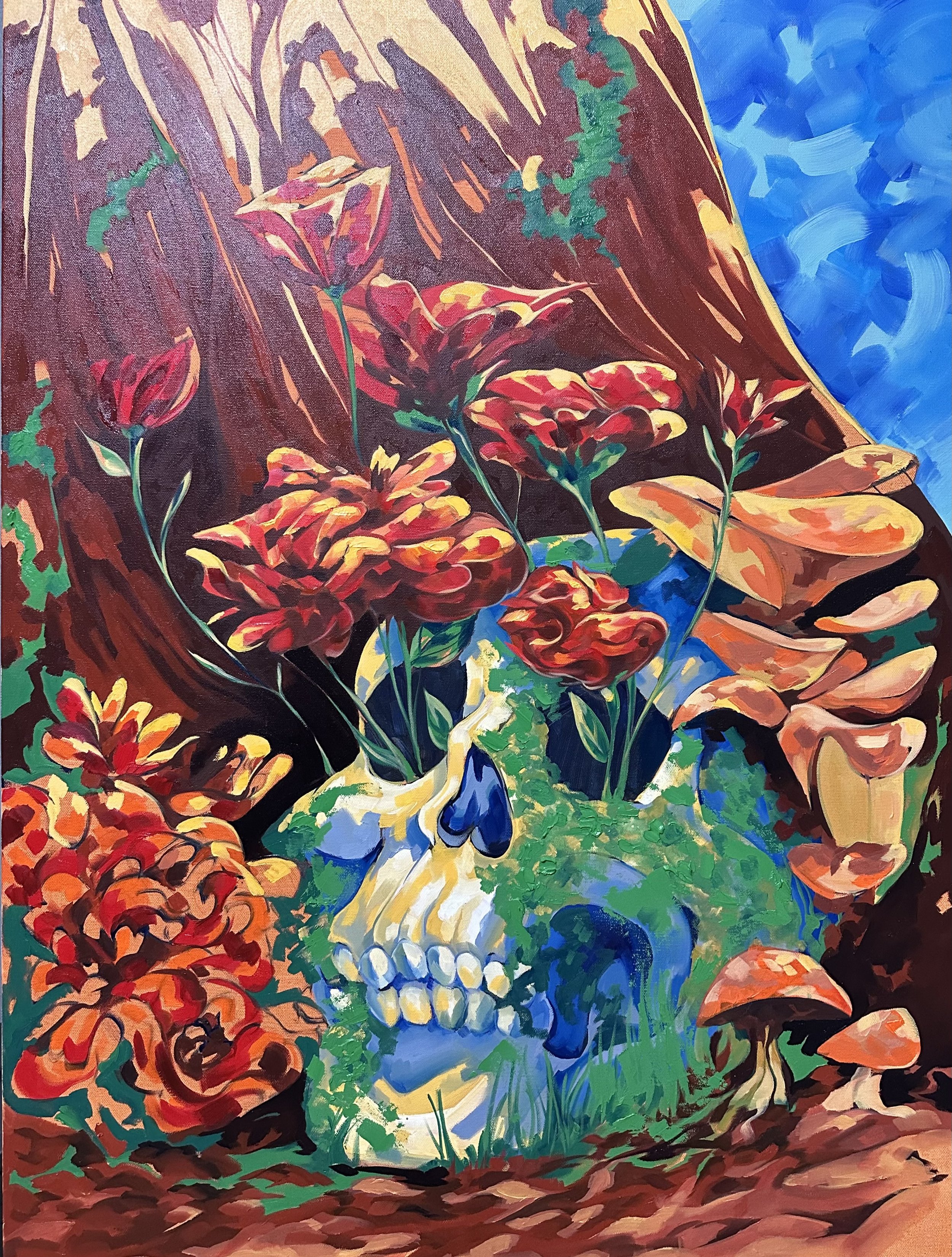The image is a vivid and detailed painting depicting a blue and green human skull positioned at the base of a brown tree. The skull, which prominently displays whitish teeth, features red and orange-shaded roses sprouting from its eye sockets. To the right of the skull, two orange mushrooms are growing. The scene is enhanced by additional flowers blooming to the left of the skull, and a lush array of green leaves adorns the tree that serves as the background. The backdrop includes hints of a blue sky, visible through the tree branches. Moss appears to be growing on and around the skull, adding to the eerie, horror-themed setting.